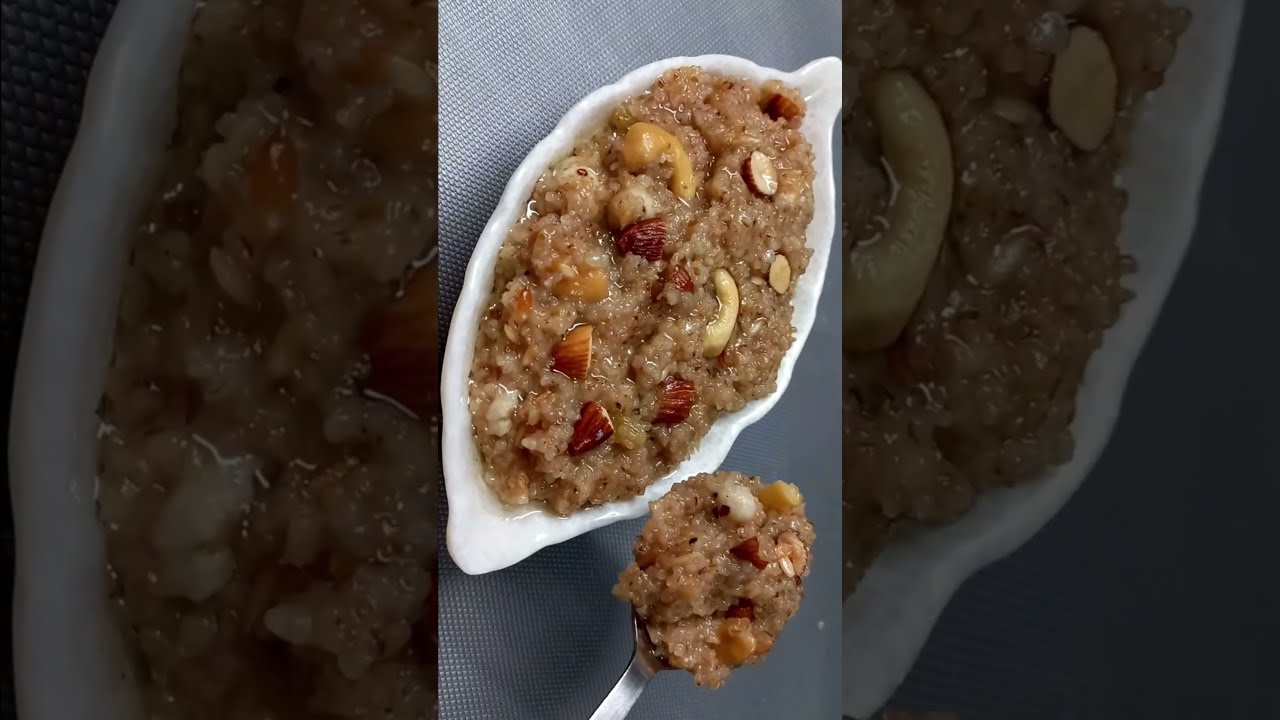The image is a detailed photograph of a unique food presentation, likely oatmeal or a similar porridge, with a rich, moist texture and adorned with an assortment of nuts. The dish is contained in a distinctive, white, leaf-shaped bowl that has a textured, uneven edge, reminiscent of a leaf or clamshell. The oatmeal, brown in color and speckled with hints of cinnamon, features an array of nuts including halved almonds and whole cashews, adding both visual and textural interest. In the lower portion of the image, a silver spoon, positioned diagonally, holds a generous scoop of this nut-studded oatmeal, echoing the contents of the bowl. The central image sits atop a grey backdrop that appears to be a tablecloth, flanked by an enlarged, blurred version of the same image on both the left and right sides, creating a framed effect for the focal dish. The entire setup rests on a white tablecloth, adding a crisp contrast to the earthy tones of the oatmeal.